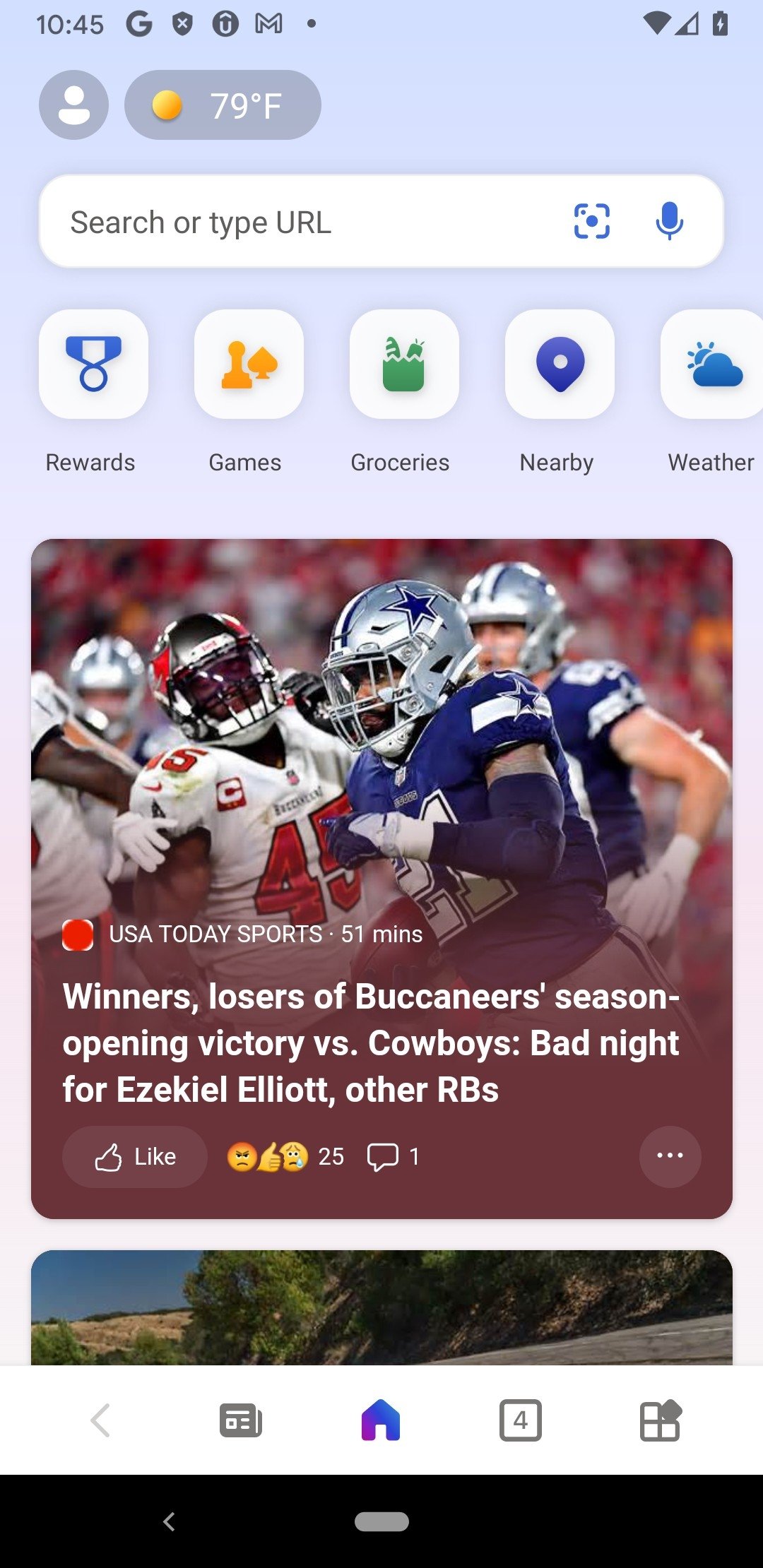A screenshot captures a person's smartphone display at 10:45 AM. At the top of the screen are various icons including Google, Google Mail, Wi-Fi, cellular coverage, and battery status. A small gray circle with the white silhouette of a person lies next to an oblong widget displaying the current weather: 79°F with a sun icon.

Below the weather widget is a search bar labeled "Search or type URL." Further down, four categorized icons are visible: "Rewards" with a blue medal icon, "Games" featuring a chess piece and a spade, "Groceries" depicted with a green grocery bag containing a baguette and a carrot, and "Nearby" indicated by a blue location pin. Additionally, "Weather" is represented by a blue cloud and a sun partially obscured behind it.

A photograph of a football game in progress is prominently displayed, captioned by USA Today Sports. It indicates it was uploaded 51 minutes ago and summarizes the winners and losers of the Buccaneers' season-opening victory against the Cowboys. Commentary includes a note on a bad night for Ezekiel Elliott and other running backs. Interaction emojis under the post include an angry face, thumbs up, and crying face, with a count of 25 reactions and one reply. Partially visible at the bottom of the screenshot is a fragment of another photograph, hinting at an outdoor scene.